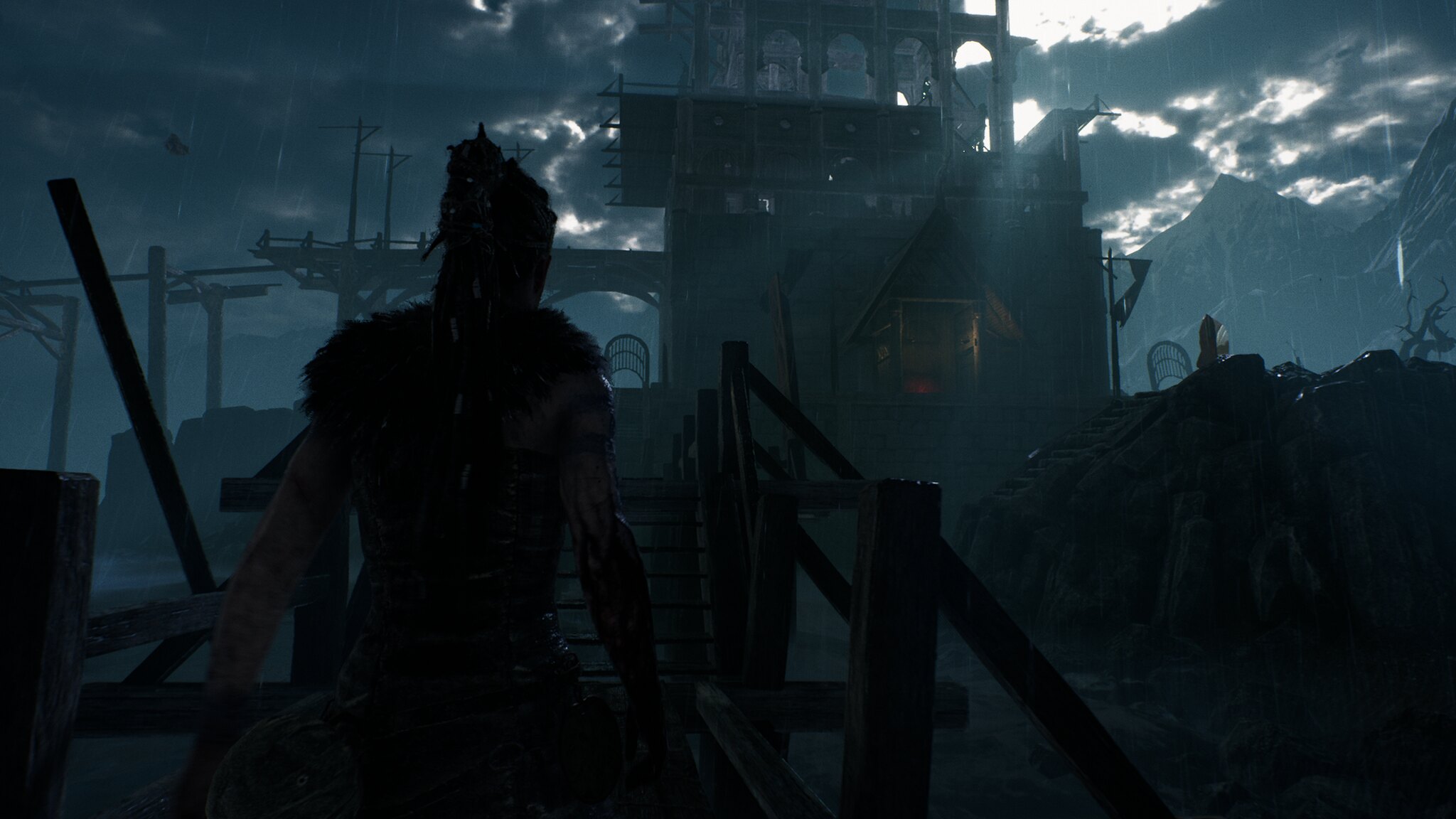The image is a dark and atmospheric 3D rendering, possibly concept art or a cinematic screenshot from the game Hellblade: Senua's Sacrifice. The setting is steeped in Norse mythology, featuring the schizophrenic protagonist, Senua, on her journey through a rainy, mountainous region to save her husband’s soul. Central to the composition, Senua stands in a fur outfit with a long braided ponytail, carrying the bagged head of her husband. Her right hand, marked by a blood curse from her underworld journey, grips the handrail of a wooden stairway that transitions into a bridge. She is making her way towards an old, partly stone building with a triangular canopy at the entryway. This building, which has visible windows and an archway through which the sky can be seen, is flanked by modern structures resembling telephone poles made of wood. Despite the rain and the dark, cloudy sky, a faint light peeks through, casting a subtle glow on the scene.